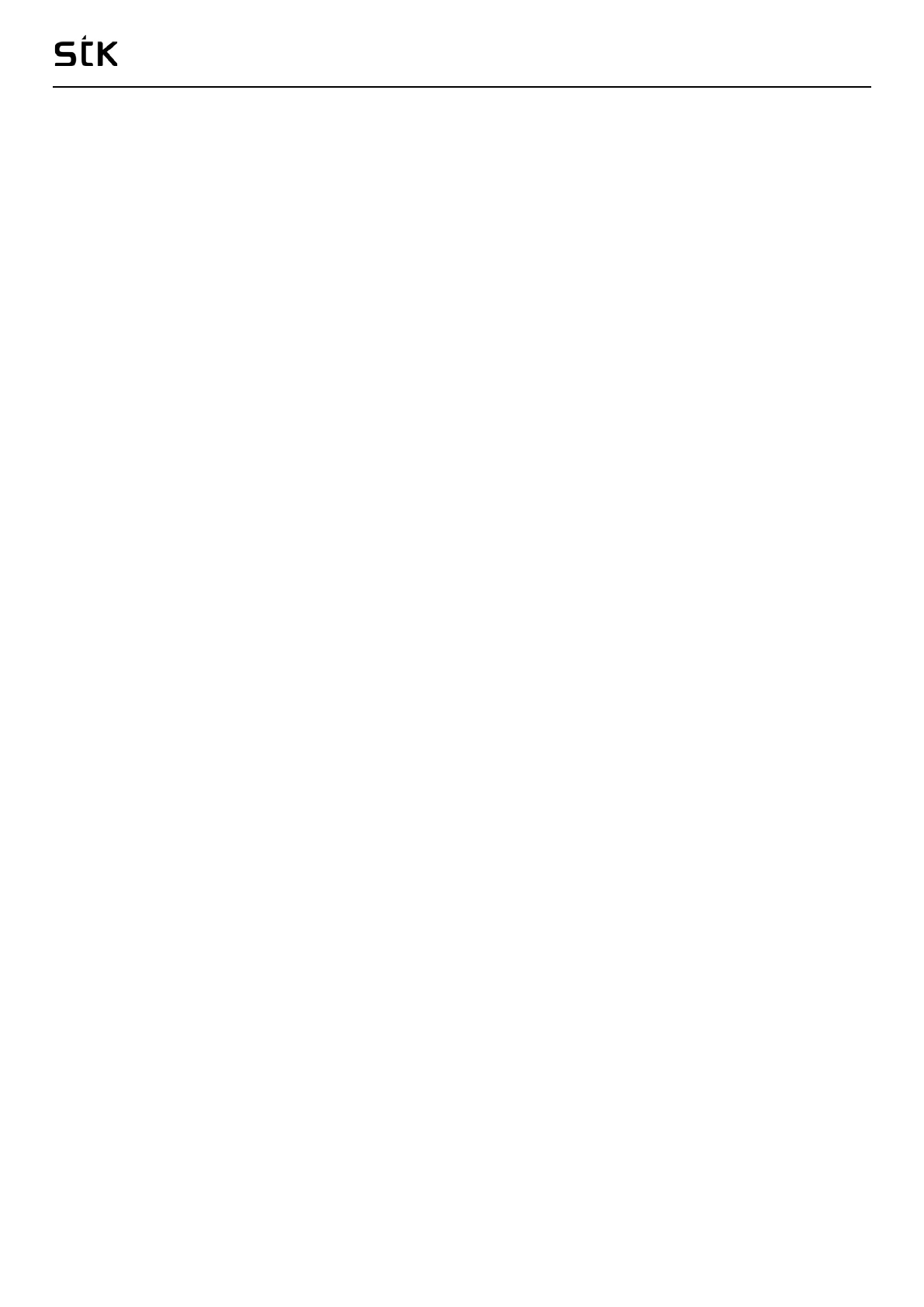The screenshot features a clean white background with a horizontal, purplish-gray line situated at the top of the page. Above this line, there are three text labels displayed in different shades of blue: "SCK Blue" in a light blue hue, "blue" in a standard blue color, and "dark blue" in a deeper shade of blue.